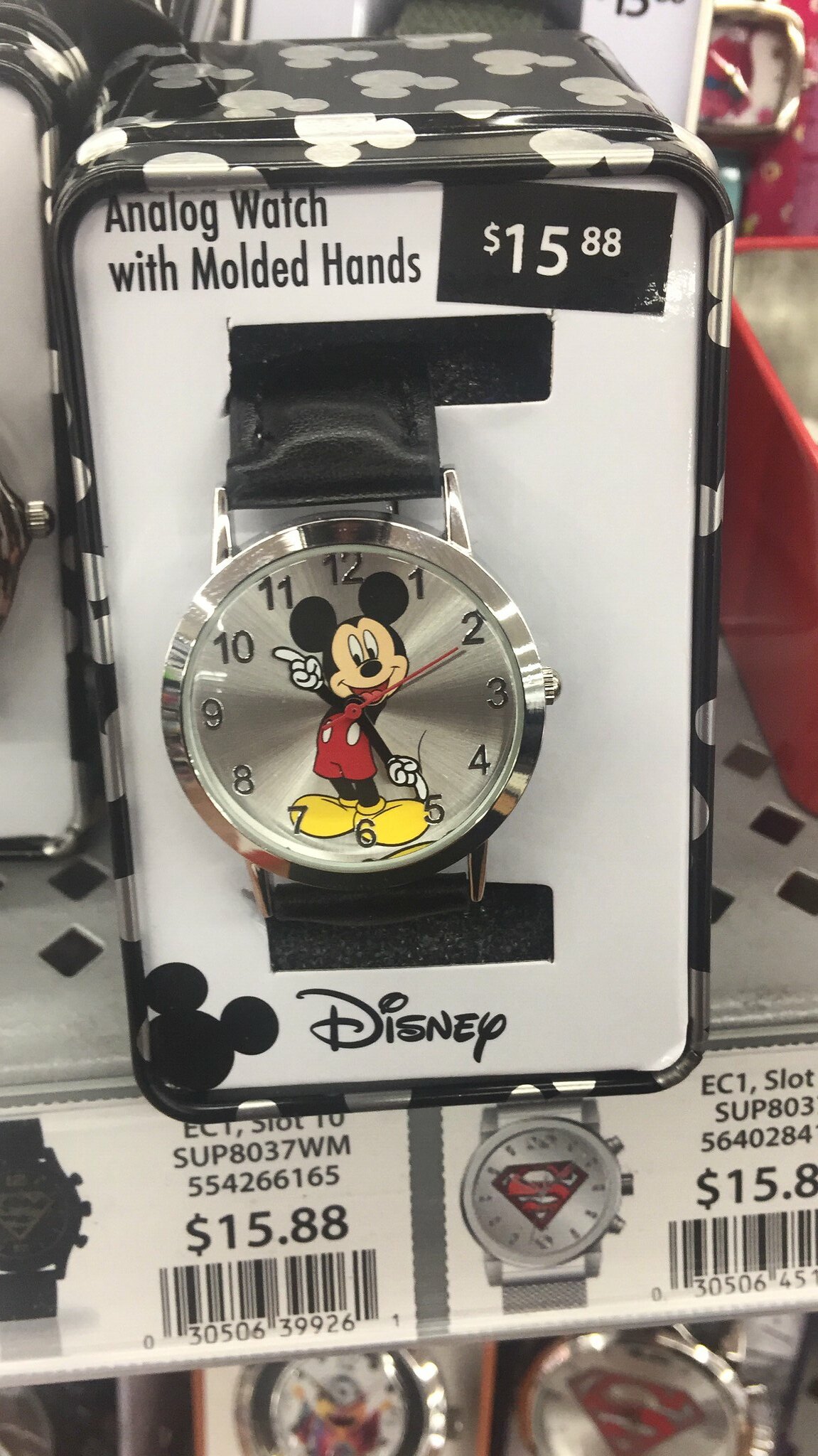This vertically-oriented rectangular image showcases a Mickey Mouse Disney watch, which is on sale and prominently displayed on a store shelf while still in its original packaging. The watch is priced at $15.88, as indicated on a black sticker with white text located in the upper right-hand corner of the packaging. Above, there is a description in black writing that reads "Analog Watch with Molded Hands." 

The background of the image is white, making the watch and packaging stand out clearly. The watch itself is securely set in a holder, highlighting both its face and band through the clear packaging. The face of the watch is silver, with matching silver casing surrounding it. Black numbers mark the hours, and the iconic Mickey Mouse is featured on the face, with his arms serving as the watch hands. The time displayed is 10:25, with the hour hand pointing at the 10, the minute hand at the 5, and the second hand at the 2.

At the bottom of the packaging, the word "Disney" is printed, along with a pattern of white Mickey Mouse heads against a black background. Each head is represented by a large circle for the face and two smaller circles for the ears.